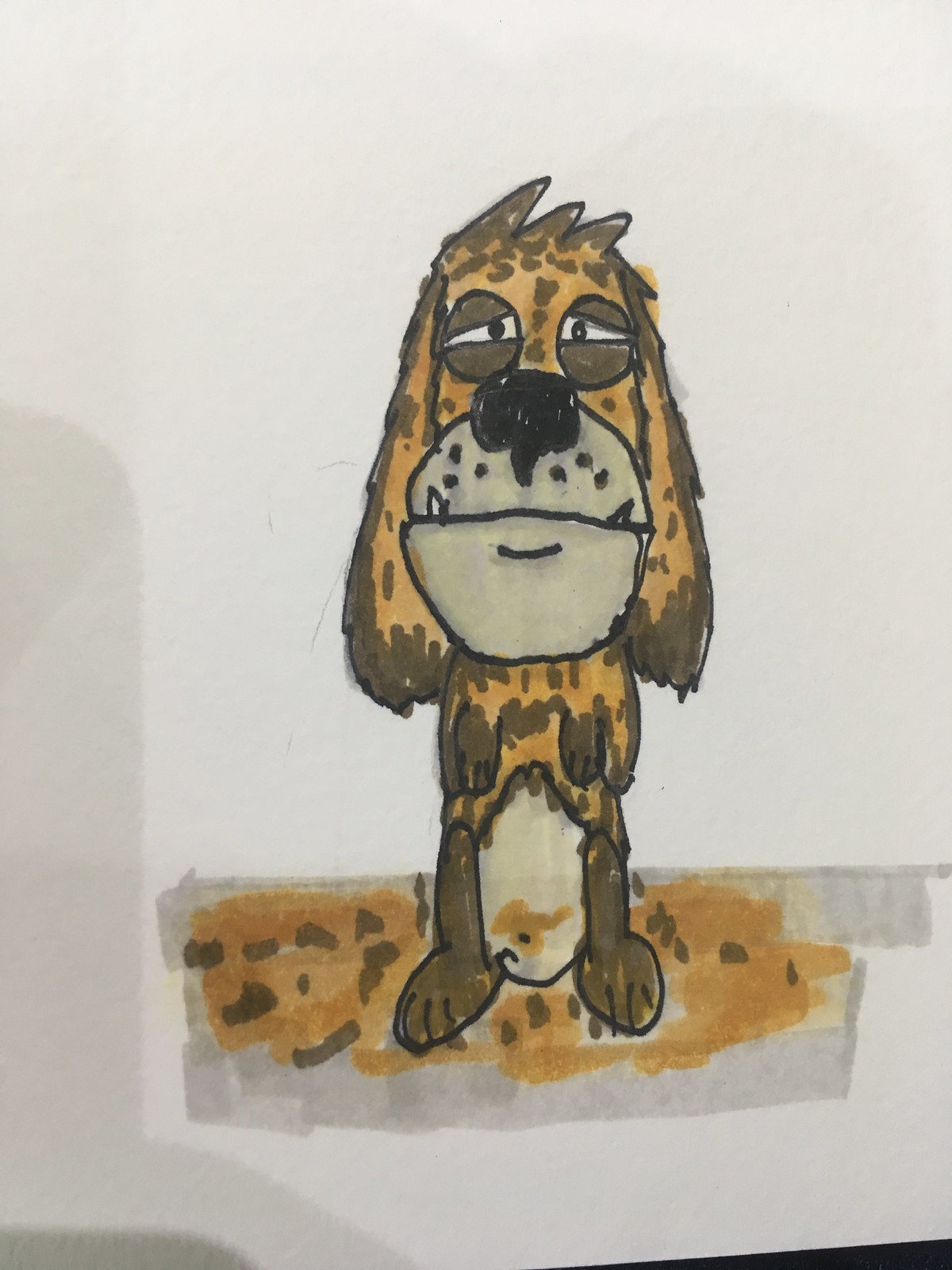This is a detailed color marker illustration on a white sheet of paper, showcasing a cartoon-style dog. The dog, characterized by its light and dark brown as well as dark orange hues, stands prominently in the center of the image. With a combination of tan and off-white accents, it displays a distinct look with its dark brown eyes peering toward its black nose, adorned with freckles. The dog has an elongated face and long floppy ears that drape down to its neck. Its small mouth, highlighted by a couple of visible canine teeth, further adds to its cartoonish charm.

The canine is depicted standing on its hind legs, with tiny paws near its neck area and larger paws supporting its stance. Its underbelly is white with intricate dark orange details, standing atop a slightly detailed ground composed of dark orange, dark brown, and light gray patches, suggesting mud. This placement enhances the overall scene, making the dog appear to be amidst a muddy environment.

Shadowing adds depth to the illustration, with a noticeable shadow cast from the left side, possibly from an iPhone used to capture this drawing. The dog's eyes, a mix of round and triangular shapes with tiny black pupils, show a sad and confused expression, further emphasized by slanted eyelids. This expressive face, combined with its dripping mud-covered appearance, evokes a sense of bewildered innocence similar to cartoon characters like Snoopy.